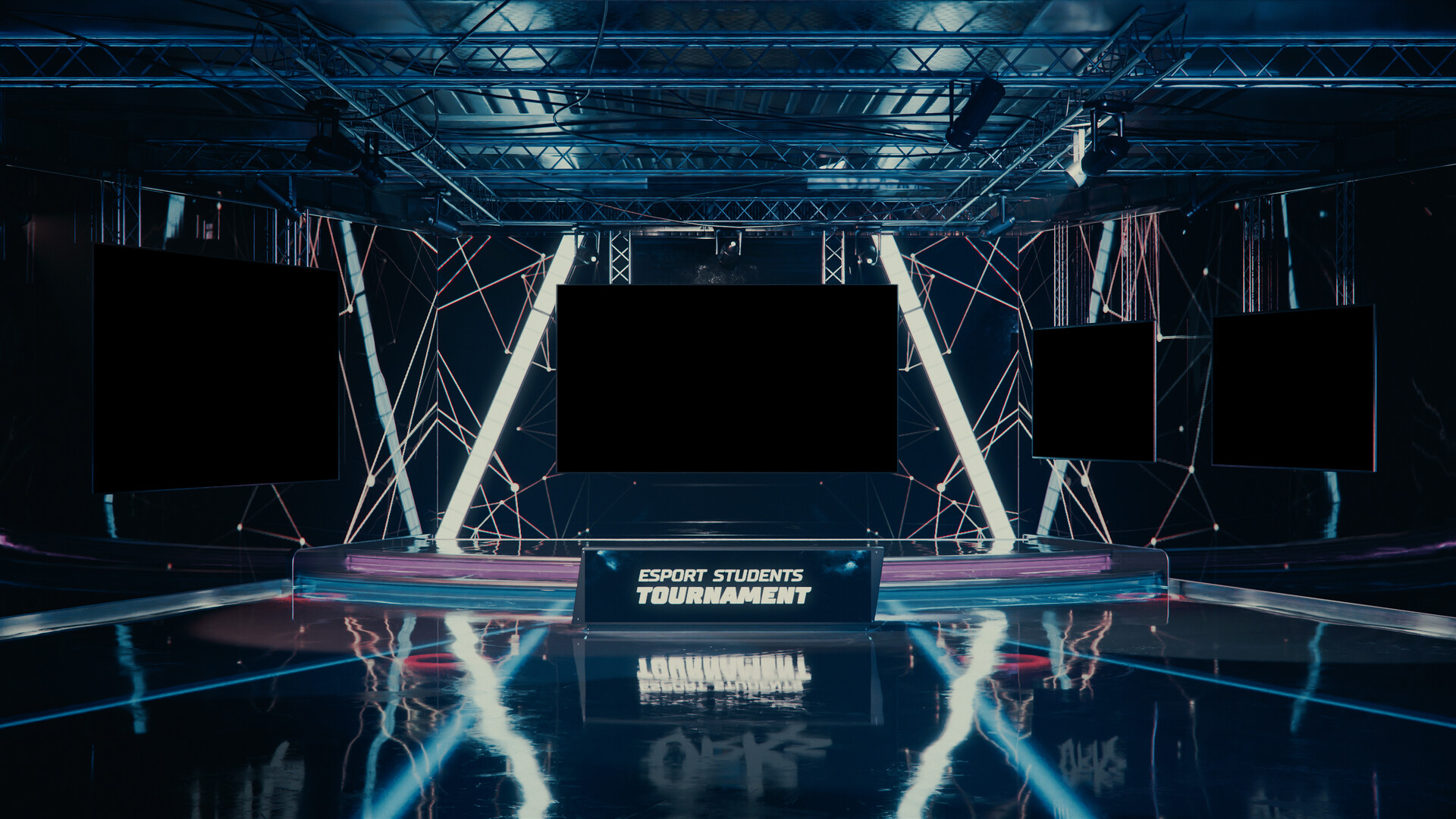This photograph, taken indoors, depicts an empty stage area in what resembles a TV studio. Central to the image is a large, non-operational black screen flanked by three other black screens—one to the left and two to the right. Below the central screen, a glowing white banner with italicized text prominently reads "Esports Students Tournament." The background is dark blue, adorned with various lights and wires, alongside a print set behind the monitors, contributing to an industrial aesthetic. Positioned below the banner are two steps, lined with unilluminated blue and pink lights—blue on the bottom step, pink on the top. The stage’s lighting, some of which is a light blue casting a faded glow on the ceiling, reflects on the polished floor, creating a vivid interplay of colors. The overall scene, awaiting activity, evokes a sense of anticipation for the forthcoming esports event.